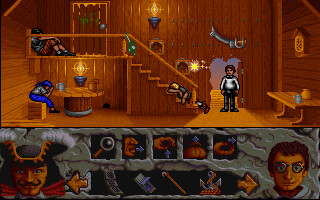This color photograph captures a computer game screen showcasing a vibrant scene. The bottom third of the image displays a gray rock with square holes cut into it, each containing various objects. On either side of the rock formation, two faces are visible: the one on the right depicts a man with brown hair and glasses, while the one on the left shows a man with black hair wearing a pirate's hat.

Above this rocky terrain, the interior transitions into a warm, golden-brown wooden setting. The entire area, including the walls, floor, staircase, and tables, is crafted from this wood. A doorway on the left lets in a stream of light, creating a brighter spot in that part of the scene. Standing in the doorway is a man with brown hair, dressed in a white shirt and black pants.

In the middle ground, a man is seated at a wooden table, adorned in a blue scarf, white shirt, and blue pants. Just above him, another man is positioned similarly on a staircase, dressed in brown pants, a white-gray shirt, and sporting dark hair. The detailed setting and character design suggest a rich narrative within the game environment.